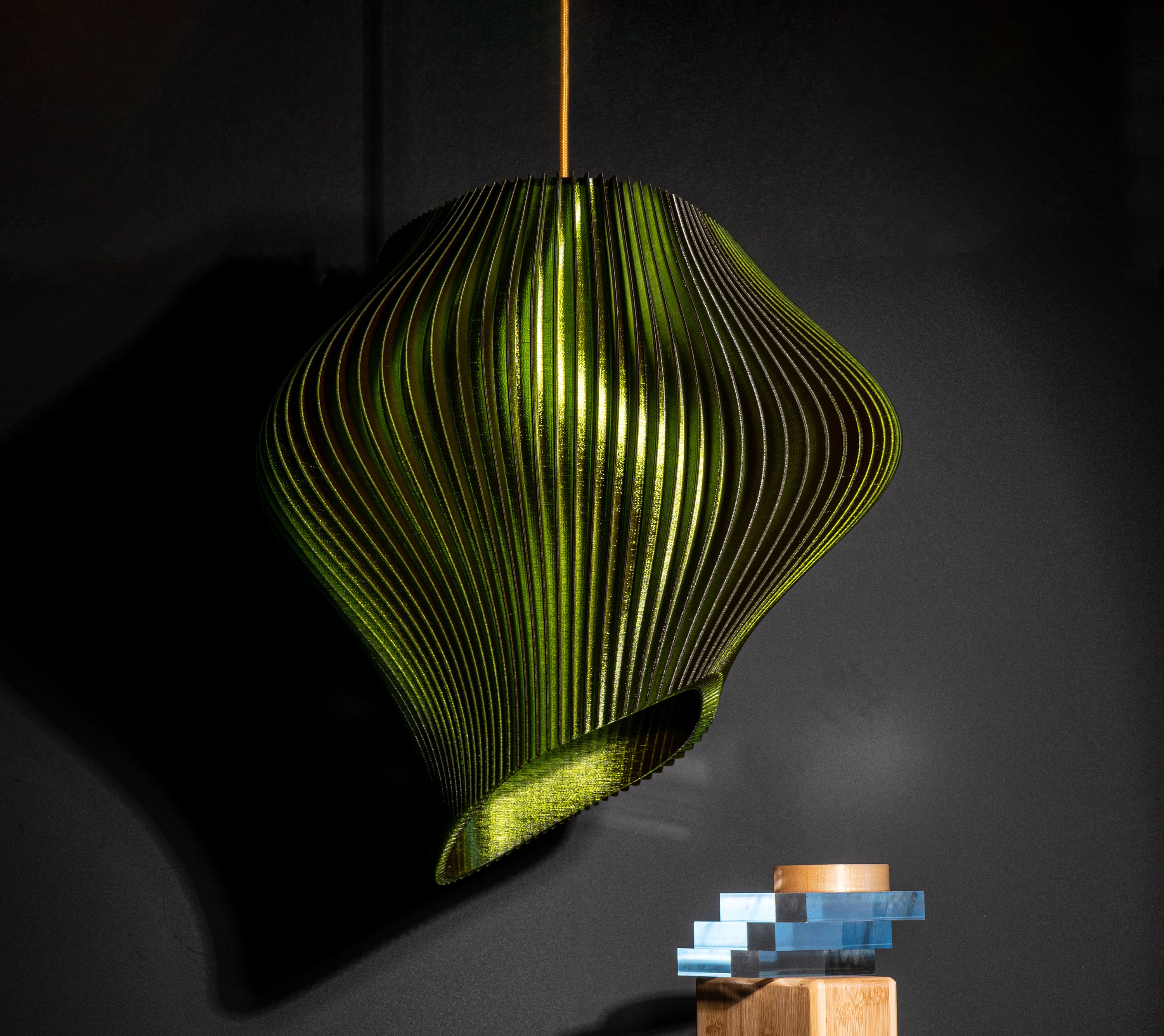The image showcases a vibrant green metallic lamp with a distinctive curvy design, set against a dark charcoal gray marbled background interspersed with dark brown hues. The lamp is suspended from the ceiling by a striking orange cord. The lampshade itself has a unique shape, beginning narrow at the top before flaring outwards and then tapering back in, finishing with a diagonal cut where the left side is lower than the right. The shade features prominent gold ridges and visible edges, providing a textured appearance. The photograph, taken indoors, frames the lamp as the central focus, casting a shadow to the left side of the wall. Below the lamp, slightly off-center to the right, rests a light beige wooden block adorned with three horizontally stacked blue glass rectangles, adding a touch of modern decor to the scene.